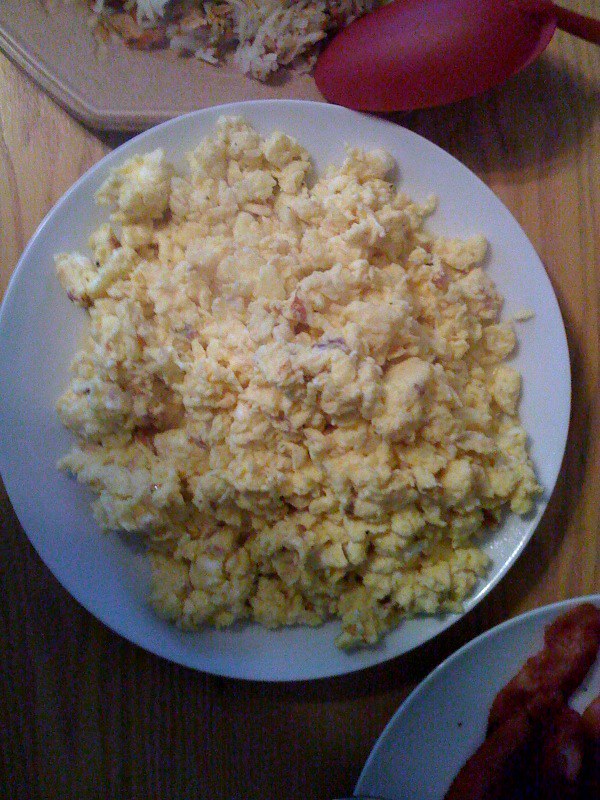This overhead photograph showcases an inviting breakfast spread arranged on a light wood grain countertop. Dominating the center is a large white plate, heaped with perfectly scrambled eggs, their golden-yellow hue flecked with what appear to be pieces of bacon or another ingredient, adding a subtle red accent. The scrambled eggs are attractively prepared, neither overcooked nor undercooked, and appear voluminous, possibly amounting to five or more eggs. In the lower right corner of the image, a second white plate is partially visible, laden with several strips of crispy bacon. At the top of the image, a cream-colored plate piled with golden hash brown potatoes occupies the frame, accompanied by a conspicuous red serving spoon. All these elements rest on a wooden table or counter, creating a comforting and hearty breakfast scene.